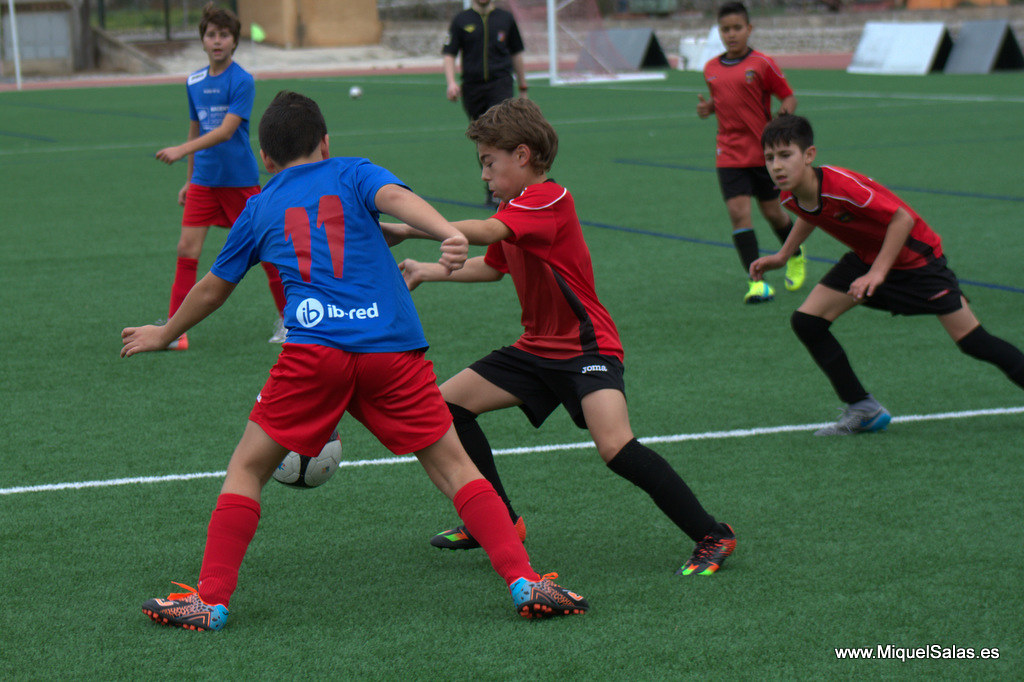The photograph captures an engaging children's soccer match, likely set in Spain as suggested by the website www.miguelsalas.es displayed in white letters at the bottom right corner of the image. The young players, appearing to be around eight to ten years old, are energetically engaged in the game. The scene is set on a meticulously maintained green field, possibly artificial turf, with distinctive white and dark blue stripes. 

The action unfolds with one child in mid-kick and others running exuberantly across the field. The game features five visible players; on the left side, two children sport blue t-shirts, red shorts, red socks, and colorful shoes. On the right, three children wear red t-shirts, black shorts, black socks, and similarly colorful footwear. The number 11 is prominently displayed on the shirt of one of the players closest to the camera.

In the background, a soccer net is faintly visible, set against the backdrop of the field. Overseeing the game is an adult figure dressed in a black short-sleeve shirt and black pants, likely a referee or coach, although their head is out of the frame. The overall ambiance suggests an outdoor setting under a slightly overcast sky, adding to the day's mild atmosphere.